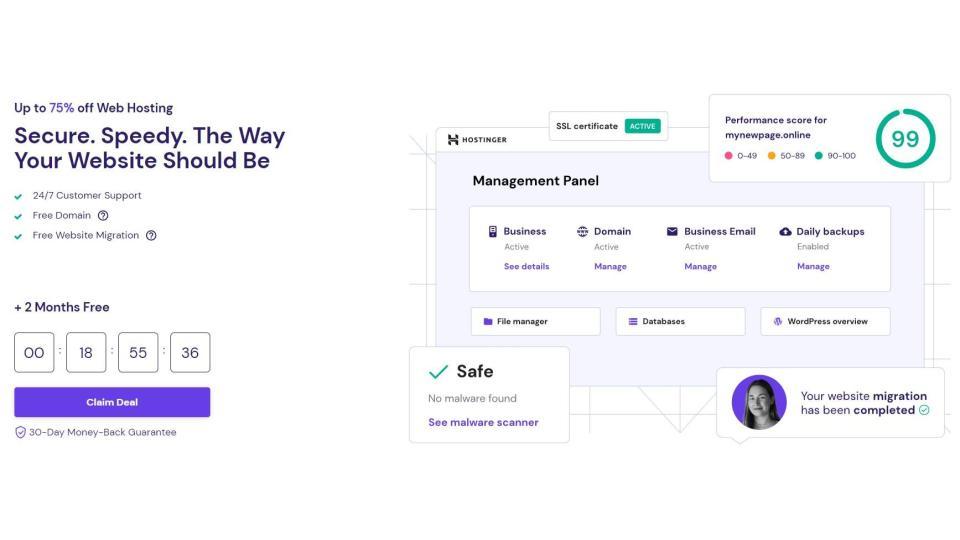The image on the screen primarily features a promotional offer for web hosting services set against a white background, making it visually borderless and expansive. The layout is notably wider than it is tall, divided neatly into two main sections.

On the left side, the text content is prominent, starting with a bold headline that reads "Up to 75% off web hosting." Below this, in larger, bold text, it captures attention with "Secure. Speedy. The way your website should be." Following this are three bulleted points detailing additional benefits:
- 24/7 customer support
- Free domain
- Free website migration

Each benefit is accompanied by a small green text box. At the bottom of this section, there's an enticing offer: "Plus 2 months free." Towards the bottom, there are four buttons, possibly indicating various options or information. Below these buttons, there is a claim offer button, and a checkbox with small print that reassures users with a "30-day money-back guarantee."

On the right side, there is an image that resembles a management panel or dashboard. This section includes various clickable options such as "Business Domain," "Business Email," and "Daily Backups," indicating the management tools available. In the upper right corner of this panel, a circled performance score reads "99," reflecting an excellent page performance metric. The lower left displays a safe icon with a green checkmark and the message "No malware found," emphasizing security. The lower right corner features a picture of a woman with a green checkmark and the message "Your website migration has been completed." Additionally, in the middle right, the presence of an "SSL Certificate" is verified with a green "Active" status.

Overall, the image serves as a comprehensive and attractive advertisement for a web hosting service, highlighting its features, security, and performance assurances.